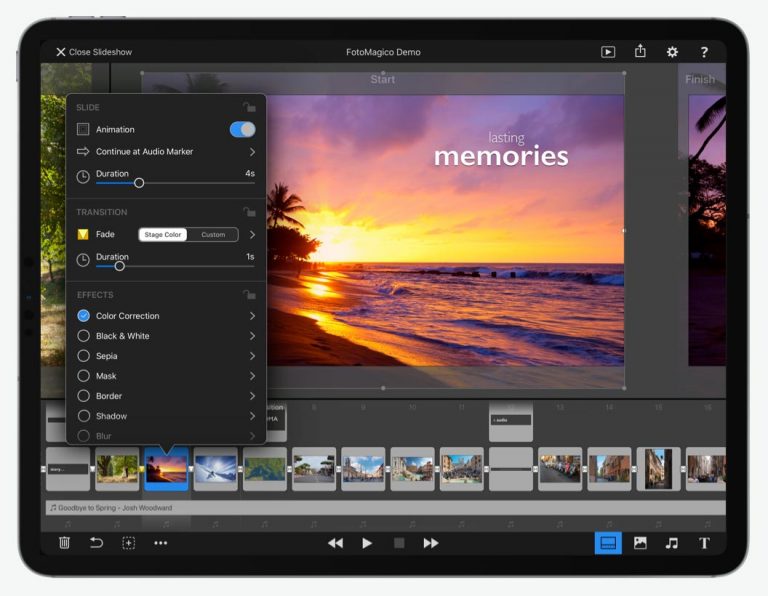The image appears to be an advertisement for a video design program showcased on a tablet. The tablet is in widescreen mode, and you can see the power button on the top right edge and the volume control buttons on the top left edge. The tablet's screen displays the user interface of the video design program, featuring a striking photo of a beach at sunset with the text "Lasting Memories" overlaid on it. The interface includes options for animation, audio maker, duration, fade, duration, and color correction.

At the bottom of the screen, there are several thumbnails of photographs or video clips arranged sequentially, suggesting the creation of home movies. Playback controls such as fast forward, rewind, play, and stop buttons are prominently visible. Additional icons for video, picture, music, and text are also present, along with delete, refresh, and a three-dot menu icon for more options. This comprehensive setup makes it apparent that the software is designed for detailed and versatile video creation and editing.